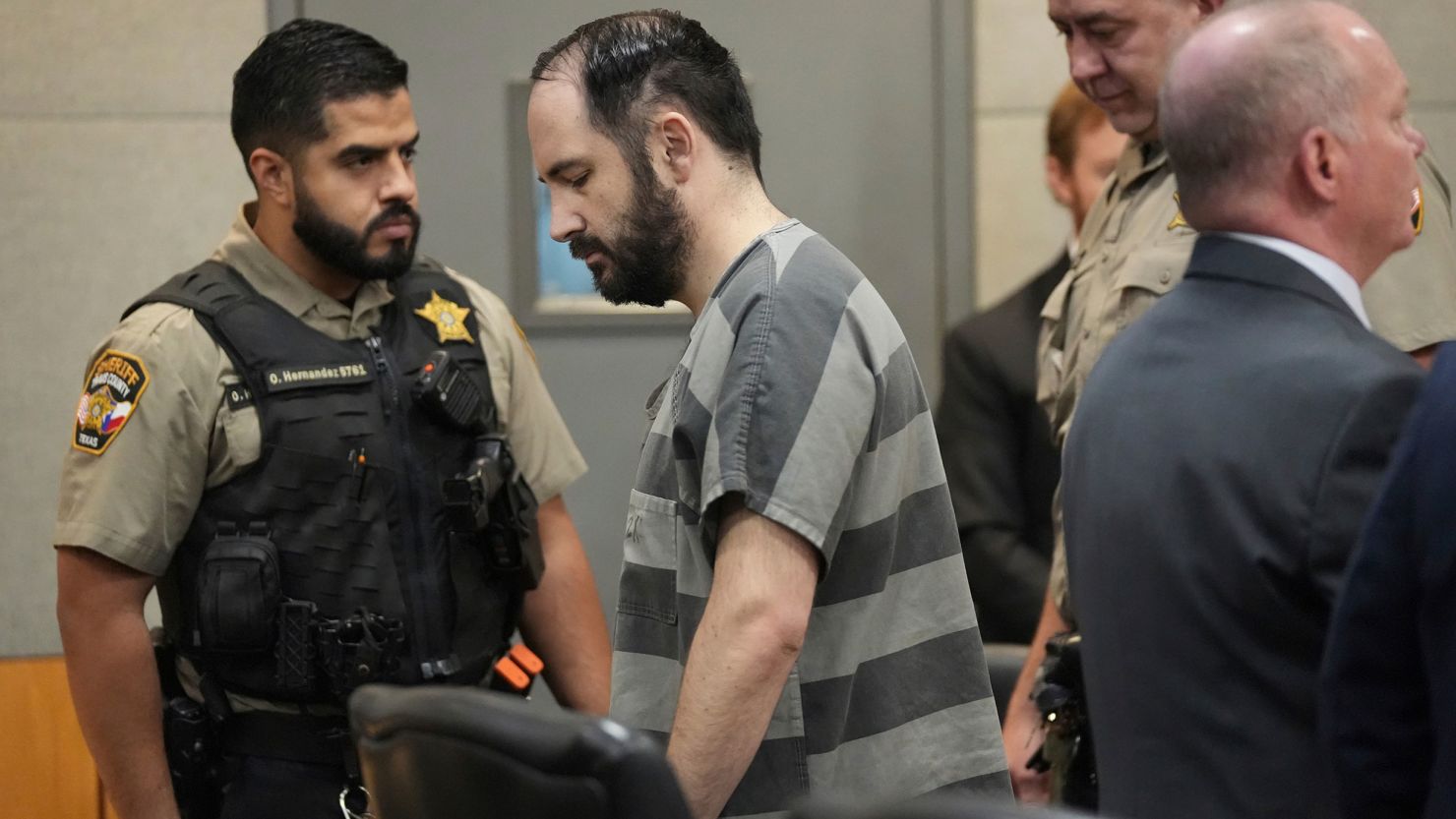In a solemn courtroom setting, a balding prisoner with a comb-over and black beard stands at the center wearing a striped shirt in bands of gray and dark gray, looking to his left. The scene captures law enforcement presence, most notably a sheriff named G. Hernandez, clad in a khaki uniform with a black tactical vest adorned with a sheriff star, a gun, a walkie-talkie, and possibly a taser. Another similarly-dressed sheriff is positioned on the right, along with two men in suits, one of whom is bald, potentially serving as the prisoner’s attorney. The background reveals the gray cement walls with orange base trim and a gray door, hinting at the institutional environment. The image is cropped to only show the individuals from about the waist up, with other people blurred or partially obscured, enhancing the focus on the central figures in this intense judicial moment.